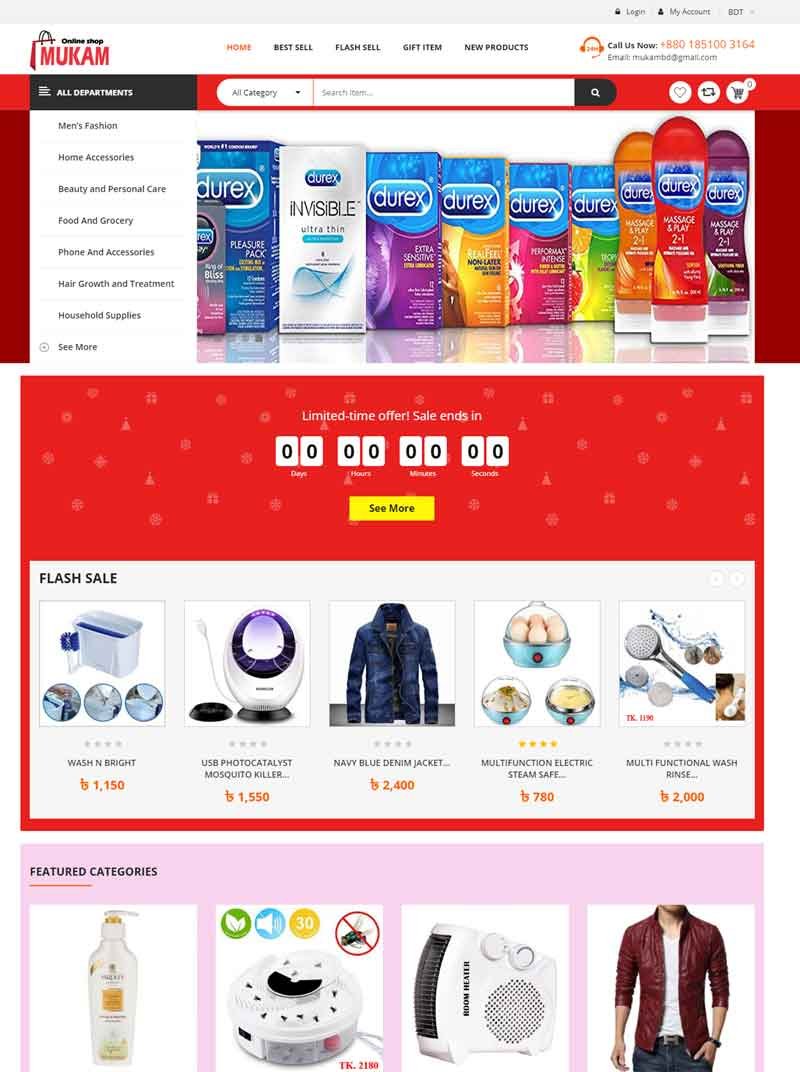The image displays an online shopping website interface with various features and items. At the top, there is a text section prompting users to "Type letters on the chart." Navigation options follow, including "Home," "Best Sellers," and "Gift Items." There is a call-to-action with the text "Call us now: 1-851-003-164" and a prompt to email. A black bar labeled "All Departments" appears, along with a category bar and a search field.

The categories listed include:
- Men's Fashion
- Home Accessories
- Beauty and Personal Care
- Food and Grocery
- Phone Accessories
- Hair Growth and Treatment
- Household Supplies

The product section displays images and descriptions of various items, predominantly Durex products such as "Durex Invisible Ultrafthin," "Durex Performance," and "Durex Massage and Play." A red bar is prominently visible in the center, adorned with various icons.

A central white banner announces a "Limited Time Offer," which states that the sale has ended (indicated by the countdown clock at zero across days, hours, minutes, and seconds). 

Several yellow rectangles label features such as "More" and "Flash Sale." Item listings follow, accompanied by pricing and ratings, including:
- ESP Photocards ($1,150)
- Mosquito Killer ($1,150)
- Navy Blue Denim Jacket ($2,400)
- Electric Steam Safe ($780)
- Multifunctional Wash ($2,000)

Further categories are indicated against a pink background. An item depicting a lotion bottle and a green circular icon, reminiscent of a heater, is also visible. Additionally, a person is shown wearing a red leather jacket.

In summary, the image captures a bustling online marketplace with vivid details about product offerings, categories, and promotional banners.